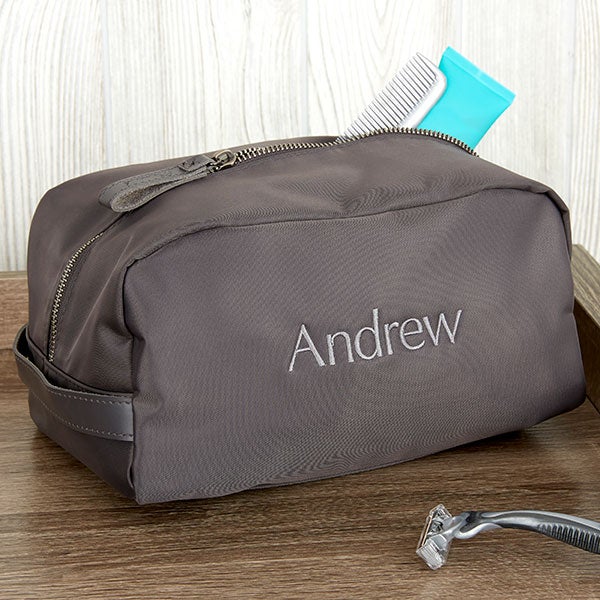The photograph showcases a square-oriented personal shaving kit centered on a wooden table with a light wooden wall as the backdrop. The focal point is a small, grayish-brown vinyl bag, specifically designed for men to hold various shaving supplies. This oval-ish square bag, resembling fake leather, features a copper-colored zipper that runs from left to right, complete with a leather pull and loop handle on the left side. Emblazoned on the side of the bag is the name "Andrew," sewn in tan-colored cloth. Protruding from the top zipper, there is a white comb and a light blue tube, while in front of the bag rests a silver razor.